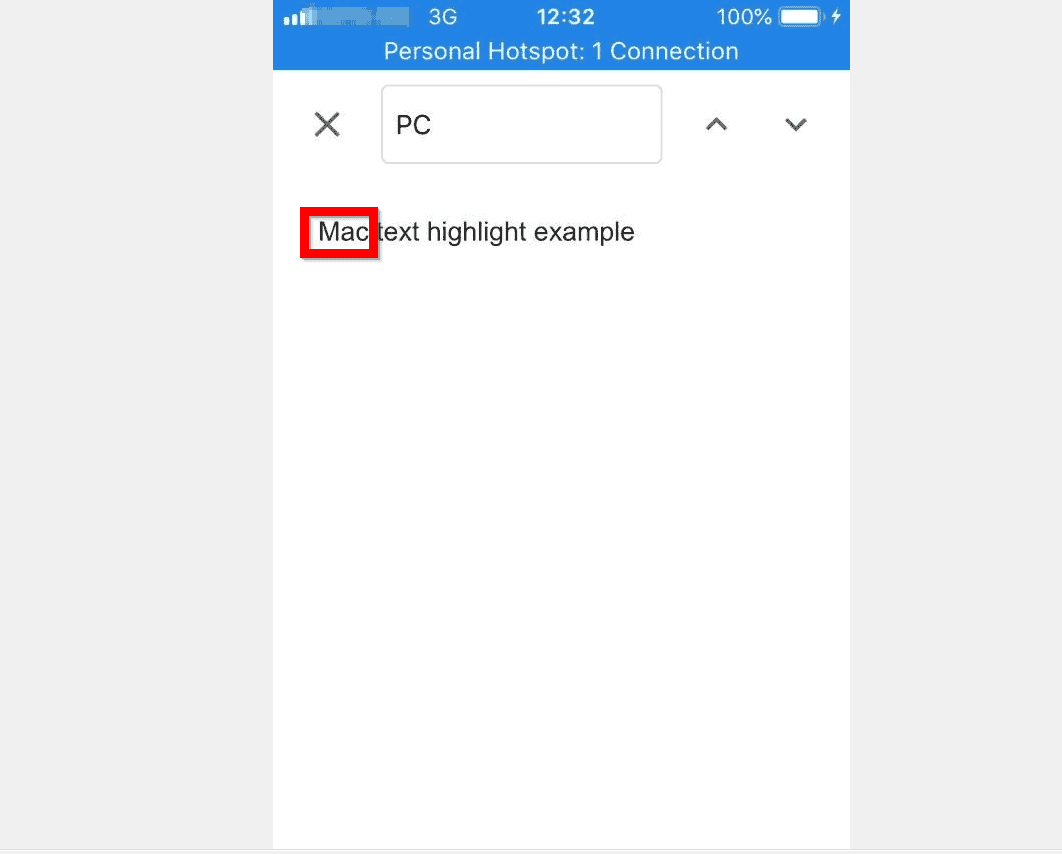A screenshot of a phone displaying the 'Personal Hotspot' option. At the top of the screen, a light blue status bar features masked signal bars, next to them the '3G' connection symbol, and the time shown as 12:32. On the right side, a fully charged battery icon with a lightning bolt indicates the phone is plugged in. Below the status bar, a field with an 'X' close button on the left and an input field labeled 'PC' on the right is visible, accompanied by up and down arrows. Underneath this is the text "Mac text highlight example", with the word 'Mac' boxed in a thick red lined square, creating a heavy drop shadow effect. The bottom section of the screenshot is largely white space. The image's background appears off-white on the sides, suggesting potential editing or formatting changes.